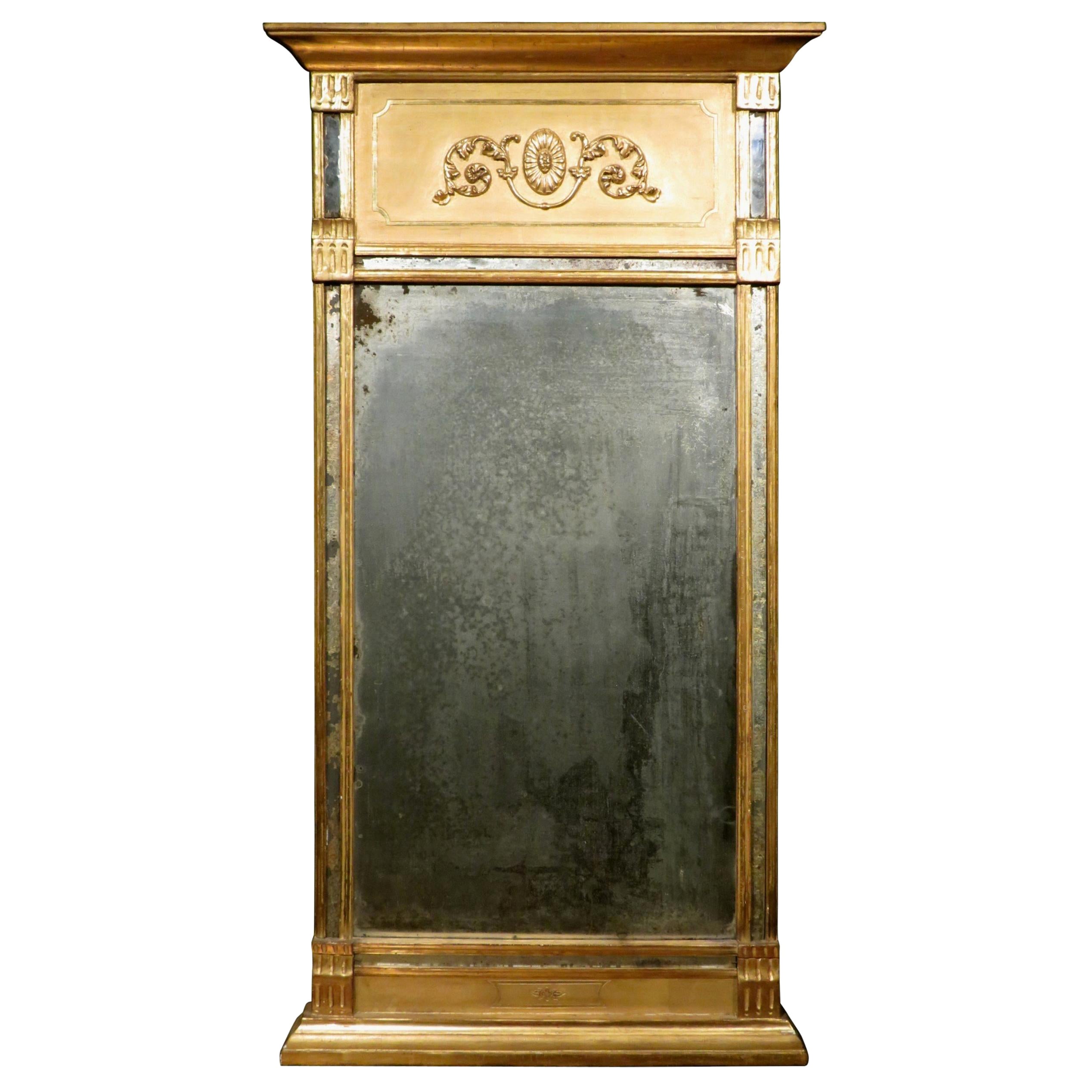The image depicts a striking antique piece, likely a decorative mirror or window frame. The entire structure is rectangular and has an ornate, golden exterior, which suggests it could be made from either wood painted gold or metal. The top section is adorned with intricate designs mimicking vines, centered around an oval shape, reminiscent of a stained glass window, but executed in a golden, possibly metallic, finish. This ornate upper part commands attention with its detailed craftsmanship.

Below this lies a large rectangular area that appears dark and aged, showing signs of rust and wear, giving it a blackish-brown hue. This surface inside the frame is mysterious; it could be a rusted mirror, an old chalkboard, or a windowpane clouded with grime, adding an intriguing, artistic element to the piece. Surrounding this central area, the golden frame extends around the edges and includes a small, rectangular emblem or logo at the top. The lower section resembles a window sill, further enhancing its architectural appeal. Overall, this piece combines a rich, decorative exterior with a rustic, weathered interior, evoking a sense of historical elegance and mystery.